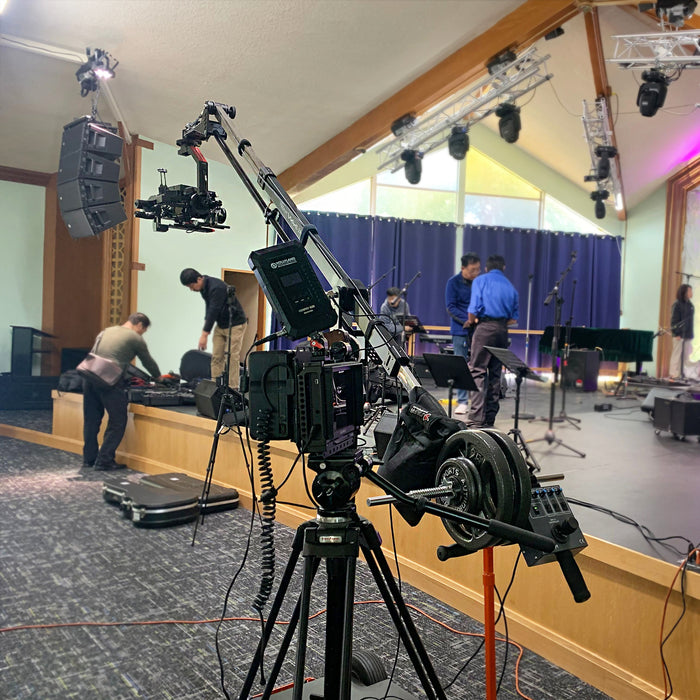The photograph captures the inside of a room featuring a performance stage set up for a musical event. The stage, located a couple of feet up on the right side of the room, has a gray floor flanked by light-colored wood sides. On the stage, several music stands intended for sheet music are visible along with black equipment boxes. A few people are either on the stage or at its side, seemingly involved in the setup. A man stands on the floor beneath the stage next to a couple of black guitar cases positioned on the left side.

The room's ceiling includes lighting rigs, while the far wall is a mix of white and wood colors. The floor exhibits a patterned gray and white surface. Prominently in the foreground is a robotic boom camera setup, comprising a complex crane mechanism with a silver and black arm extending towards the stage. Attached to this crane is a sophisticated camera rig with controls including a joystick and slider buttons, along with barbell weights serving as counterbalances. Nearby, a traditional video camera is also set up, likely part of the recording equipment. The scene appears to be an active setup for a musical performance, possibly in a church, given the presence of musical instruments and sheet music stands.